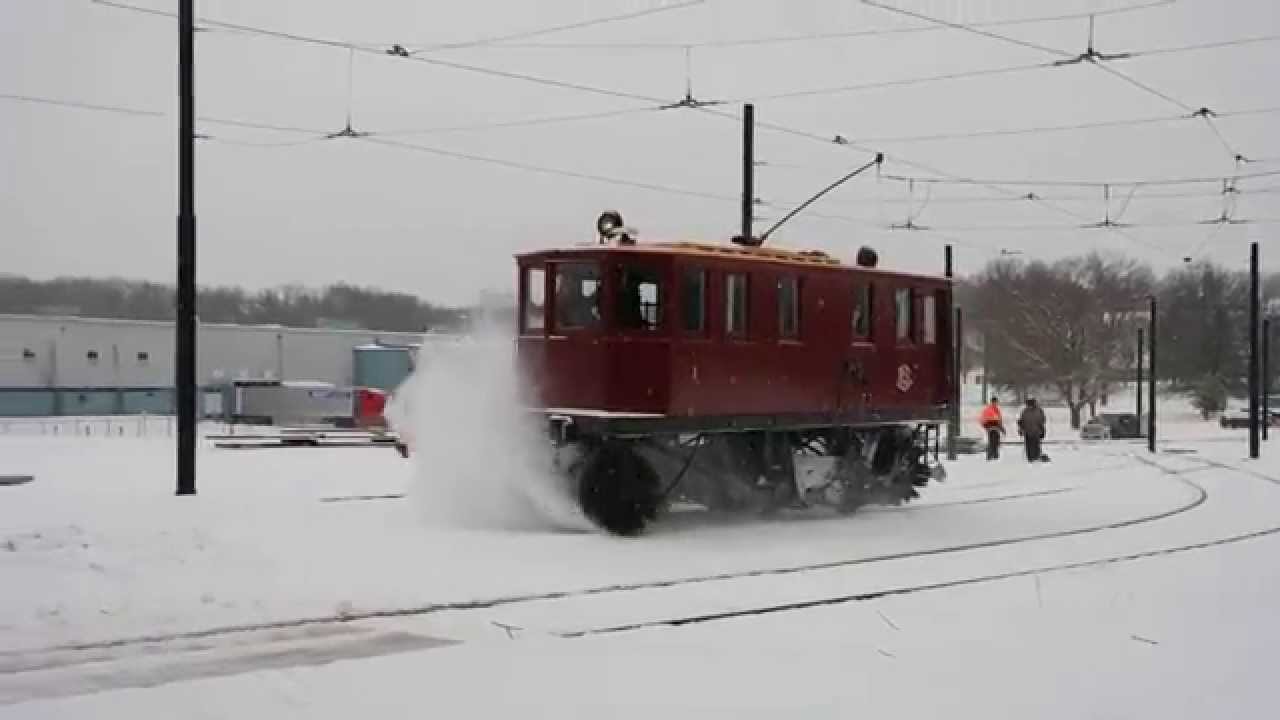In this photograph, a red electric tram with numerous windows is captured plowing through snowy railroad tracks under a bleak, white winter sky filled with clouds. Central to the image, the tram is connected to an overhead electrical grid essential for its operation. The vehicle features a distinct color scheme with a red upper body, and a black and gray bottom with visible wheels. To the right side of the photograph, two individuals—one notably wearing an orange jacket—walk near the tracks, suggesting they might be workers. On the left side, an industrial gray building and other cars are visible, adding to the urban landscape. The scene is devoid of any text or signage, emphasizing the stark, wintry environment.